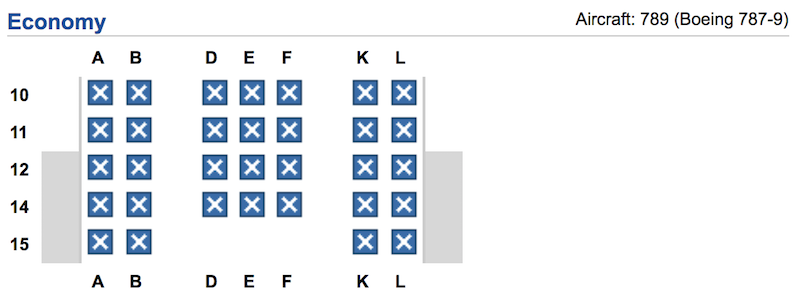This is a screenshot with a white background. In the top left corner, "Economy" is written in dark blue font. In the upper right corner, "Aircraft: 789 (Boeing 787-9)" is displayed in black font. Below this text, there's a faint black horizontal line, followed by a seating chart. 

The seating chart is labeled vertically from rows 10 to 15 in black font on the left side. Horizontally, the columns are labeled "A," "B," "D," "E," "F," "K," and "L" at both the top and bottom of the chart. 

Within the chart, rows "A" and "B" each contain five blue squares marked with white X's. Rows "D," "E," and "F" each have four blue squares with white X's. Rows "K" and "L" also each have five blue squares with white X's. 

Additionally, there are two small gray rectangles on either side of the seating chart. This chart appears to depict the seat layout of the aircraft.